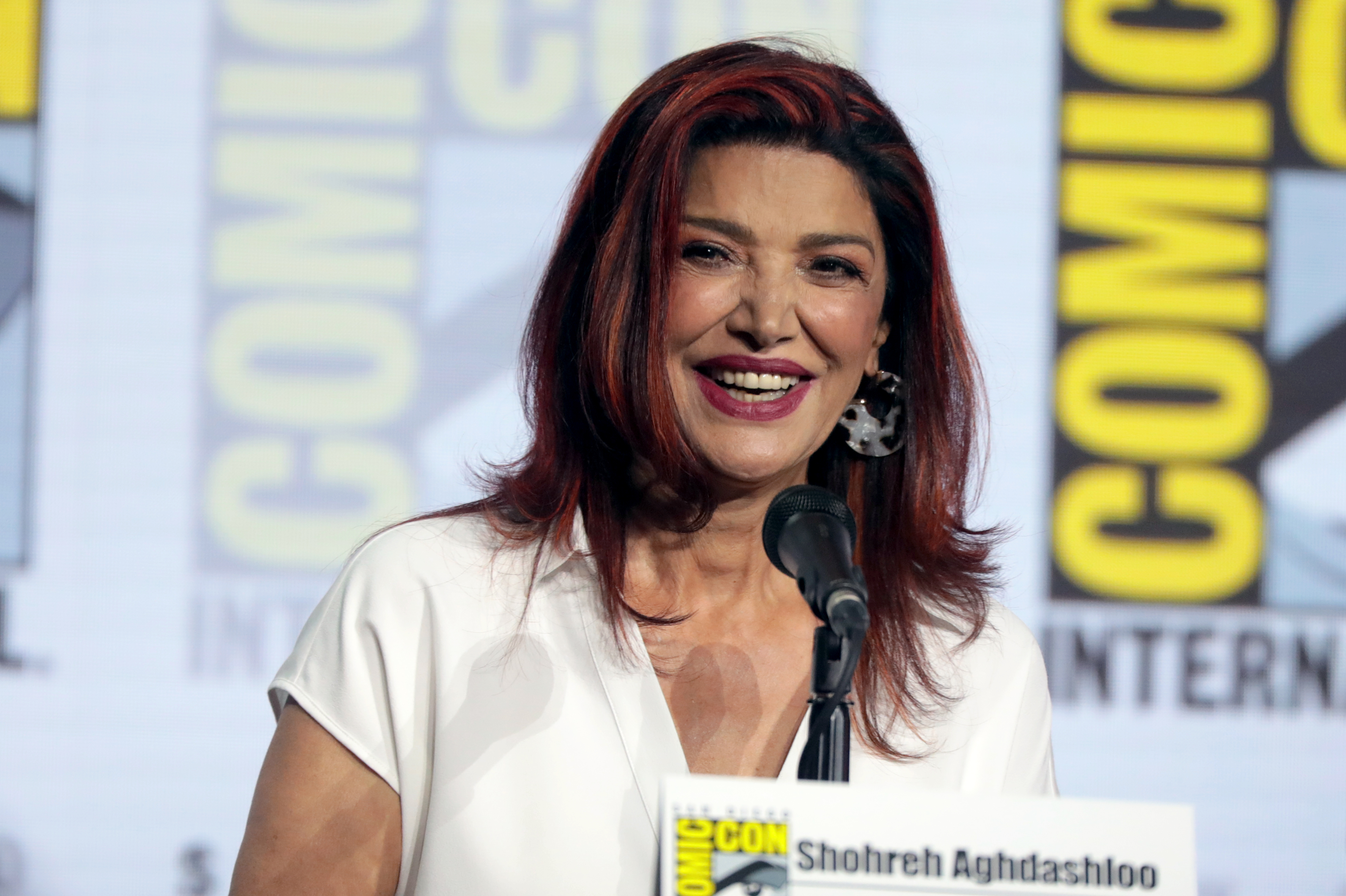The photograph features Shohreh Aghdashloo, an actress, seated at a podium during a Comic-Con event. She is in front of a white backdrop that prominently displays the Comic-Con logo repeatedly in yellow letters. Shohreh's name is visible on a standing sign with the same Comic-Con logo. She is wearing a white dress with a V-neck cut, accessorized with large, distinctive dangling earrings that feature an unusual design, likely incorporating some unique creature or insignia. Shohreh's medium-length hair is a mix of black and dark red with highlights, and she sports red lipstick. She is smiling broadly, showing both her top and bottom teeth, and is positioned in front of a black microphone, looking slightly to the left. Behind her, the Comic-Con logos and sign add context to the lively and engaging setting.